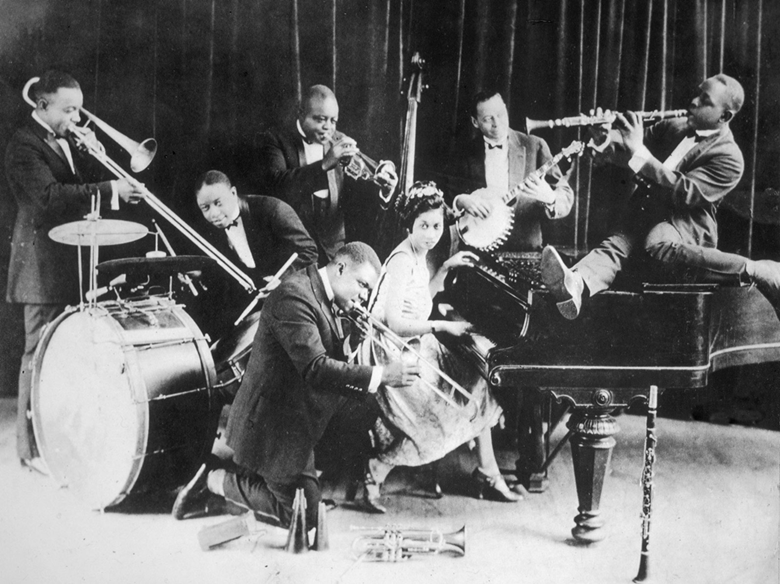This evocative black-and-white photograph, likely from the 1920s or 30s, captures a lively seven-member African American jazz ensemble. The ensemble features a striking woman at the center, adorned in a shiny cocktail dress and Mary Jane style heels, seated gracefully at a black baby grand piano. She gazes directly into the camera, one hand poised on the piano keys and the other resting atop the piano. Surrounding her are six dapper men dressed in black tuxedo-style suits with bow ties, each engaged with their instrument in various dynamic positions. Perched on top of the piano is a clarinetist, legs sprawled, playing his instrument with fervor. Kneeling beside the piano, a trombonist adds a brassy flair to the composition. In the ensemble's backdrop, a banjo player strums melodically while a trumpeter stands next to a towering stand-up bass, adding depth to the musical tableau. Completing the scene, a drummer, bent over with drumsticks in hand, prepares to set the rhythm. This carefully posed, yet vibrantly spontaneous image encapsulates the spirit and camaraderie of early jazz.